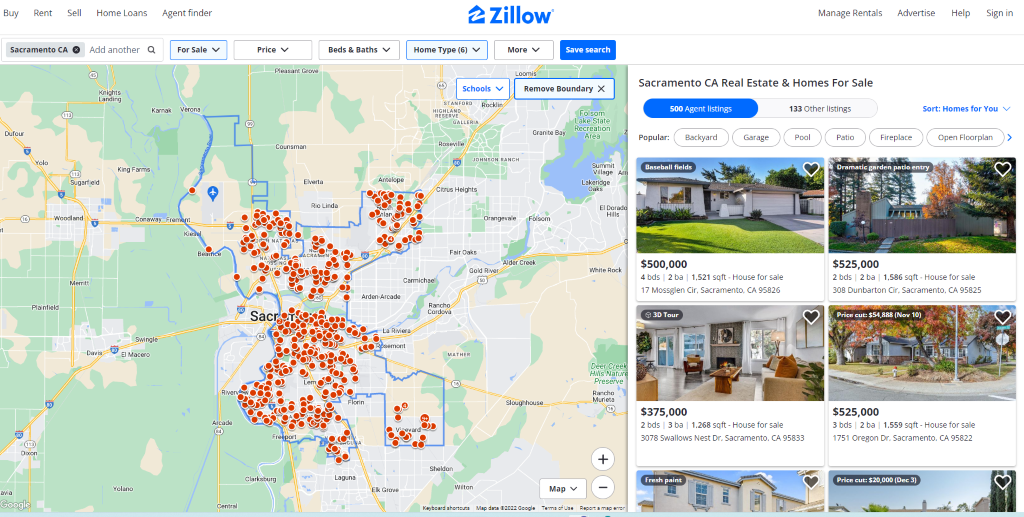Here is a cleaned-up and detailed caption for the image described:

---

This is a screenshot of Zillow's homepage. At the top center, the Zillow logo is prominently displayed in bold blue letters, accompanied by the Zillow icon—a blue house silhouette featuring a white "Z" across it. 

On the left-hand side, a gray navigation bar lists various tabs: "Buy," "Rent," "Sell," "Home Loans," and "Agent Finder." On the right-hand side, there are additional tabs labeled "Manage Rentals," "Advertise," "Help," and "Sign In."

Below the navigation bars, there are multiple search fields and filters. The first field, which is a search bar for location, shows "Sacramento, California." Adjacent to this, a dropdown menu is set to "For Sale." Following that, there are additional dropdown menus for filtering by "Price," "Beds & Baths," "Home Type" (noted with a blue indicator and the number "6" suggesting six types are selected), and "More." A blue "Save Search" button with white text is situated at the end of the filter row.

Below these filters is a map, likely of California, displaying various labeled areas such as Laguna and Sacramento Kings Farm.

On the right-hand side, the section is titled "Sacramento, California Real Estate and Homes for Sale," showcasing six property listings. The listings include:
- A four-bedroom home priced at $500,000
- A two-bedroom home priced at $525,000
- Another two-bedroom home priced at $375,000
- A three-bedroom home priced at $525,000

The image reflects an active search for real estate in Sacramento, California, utilizing Zillow's various search and filter functionalities.